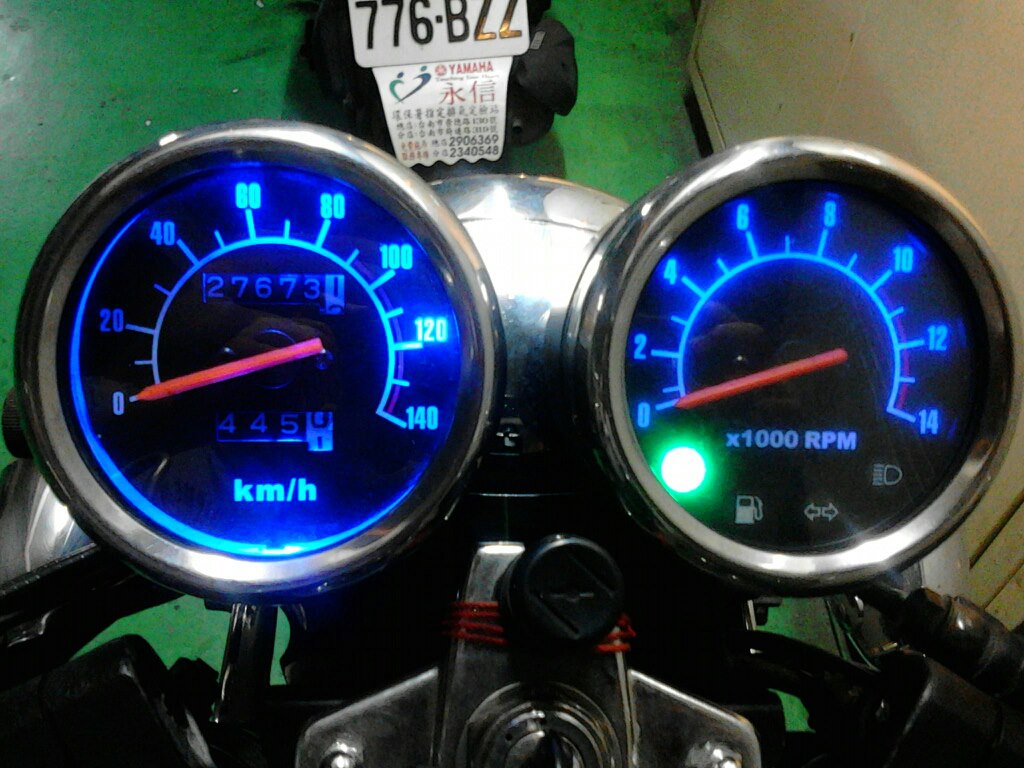A detailed close-up photograph of a motorcycle's dashboard reveals a speedometer and another gauge. The speedometer is prominently displayed with white numbers that are backlit to emit a striking blue glow. The gauge hands stand out in vivid red or orange hues. Both instruments are framed in sleek chrome, blending seamlessly with the motorcycle's overall design in this section. 

The background is entirely black, enhancing the illuminated details. A green indicator light, adjacent to the gasoline light, is visible, though its specific purpose is unclear. The surrounding area includes partial views of the handlebars and minimally the bike's surface. In the distant background, the ground, possibly a garage floor, is discernible.

The image also captures another motorcycle positioned in front, showing a partially visible license plate that reads "776B22." A Yamaha tag with additional characters and numbers dangles from the license plate, contributing to the layered composition of the photograph.